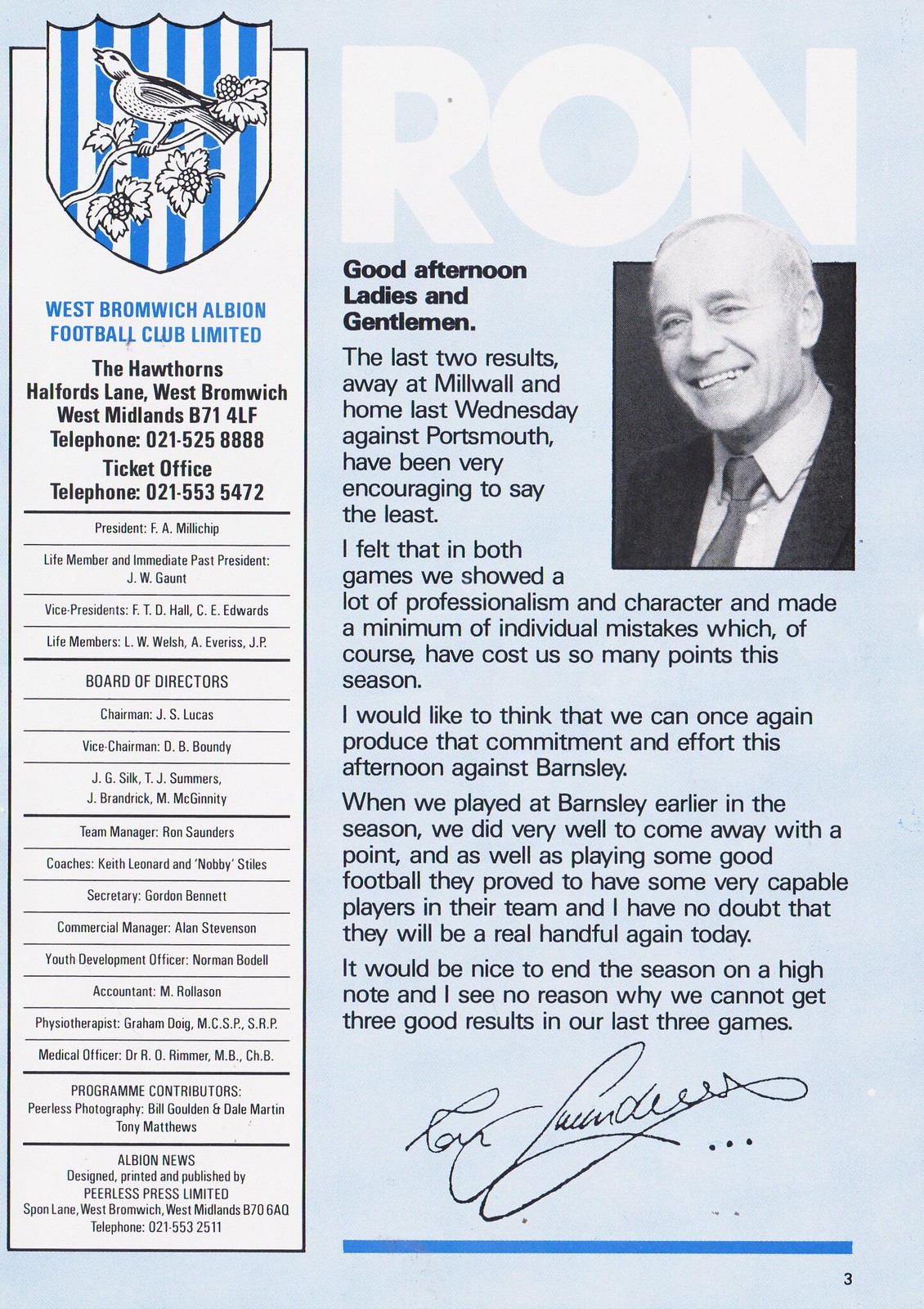A tall, rectangular image designed as a poster or magazine page features a light blue background. Dominating the left side, a white vertical rectangle with a black border presents a blue and white vertically striped shield with a bird perched on a branch at its top. Below the shield, it lists several names and the text “West Bromwich Albion Football Club Limited, The Hawthorns, Halfords Lane, West Bromwich, West Midlands, B714LF, telephone 021-525-8888, ticket office telephone 021-553-5472.” Adjacent to this, in prominent white all-capital letters, the word "RON" is displayed, followed by a bold black greeting: "Good afternoon ladies and gentlemen."

Accompanying this greeting are five paragraphs of text expressing reflection and optimism regarding recent football matches. The text details the club’s recent games - an away match at Millwall and a home game against Portsmouth - highlighting the team's professionalism, character, and minimization of individual mistakes. The narrative is an aspirational message for an upcoming game against Barnsley, emphasizing the players' efforts and the coach's optimism. This message is concluded with a signature line underlined by a horizontal blue line and a small number "3" in the bottom right corner. To the right of the name "Ron," there is an image of a smiling man, identified as Ron Saunders, likely the coach providing these insights and encouragements.